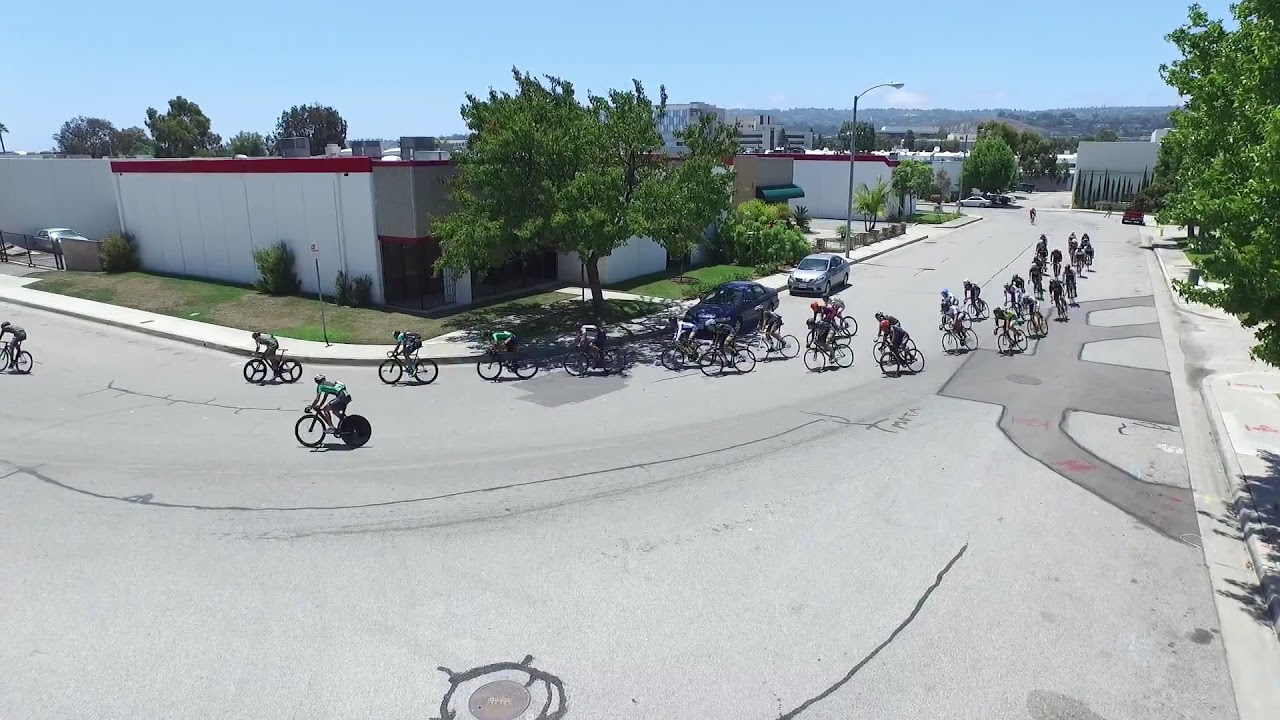This horizontally aligned rectangular photograph captures an outdoor daytime scene where a dense group of cyclists, likely participating in a race or marathon, is navigating a curve from the right towards the left side of the image. The grey paved road they are on shows signs of wear with black markings, cracks, and a manhole in the center bottom of the image. 

The setting includes a clear blue sky with a couple of small white clouds far in the distance. A white-stone building with a red trim on top and two vehicles partly hidden by the cyclists are prominent in the center. This structure, resembling an industrial warehouse, is situated on the left with some grass patches and greenery around. Trees punctuate the scenery, with one full green tree on the sidewalk corner and another partially visible in the upper right corner. 

The backdrop features a green hillside under the cloudless sky, emphasizing the outdoor location. The road, flanked by a sidewalk on its right side, appears aged and experienced with traffic. There are approximately 20 to 30 cyclists, all wearing helmets, and although it's unclear if they are in uniform, their figures blend into the vivid landscape of green, brown, white, grey, black, and various shades of blue and green.